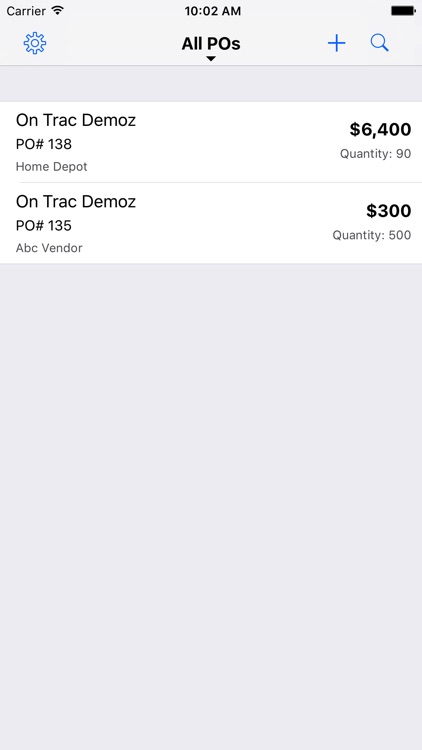A detailed caption of the image reads as follows:

---
The image is a high-quality screenshot of a settings menu with a white-gray background and black font. At the top of the screen, the word "Carrier" is displayed prominently. Also visible are a Wi-Fi icon resembling a funnel or tornado, the time "10:02 a.m.", and a fully charged battery icon. Below these, a blue cogwheel icon is present. 

The menu title "All P.O.s" is in bold black font with a drop-down arrow next to it, indicating that it can be clicked. To its right are a blue plus sign and a blue magnifying glass icon. 

Further down, the screen displays a light-gray strip, followed by more black font text. It reads "On Track Demos with a Z," followed by "P.O. number 138, Home Depot, $6,400, quantity 90." A thin gray line separates this entry from the next.

The following line also reads "On Track Demos with a Z," but this time the details are "P.O. number 135, ABC Vendor, $300, quantity 500." The prices are in bold black font, and the quantities are in a paler gray font.

Towards the bottom of the screen, there is a large, empty gray box. The entire screenshot is of excellent quality, with no pixelation or blurring, making the text bold and easy to read. No other images or notable elements are present on the screen.